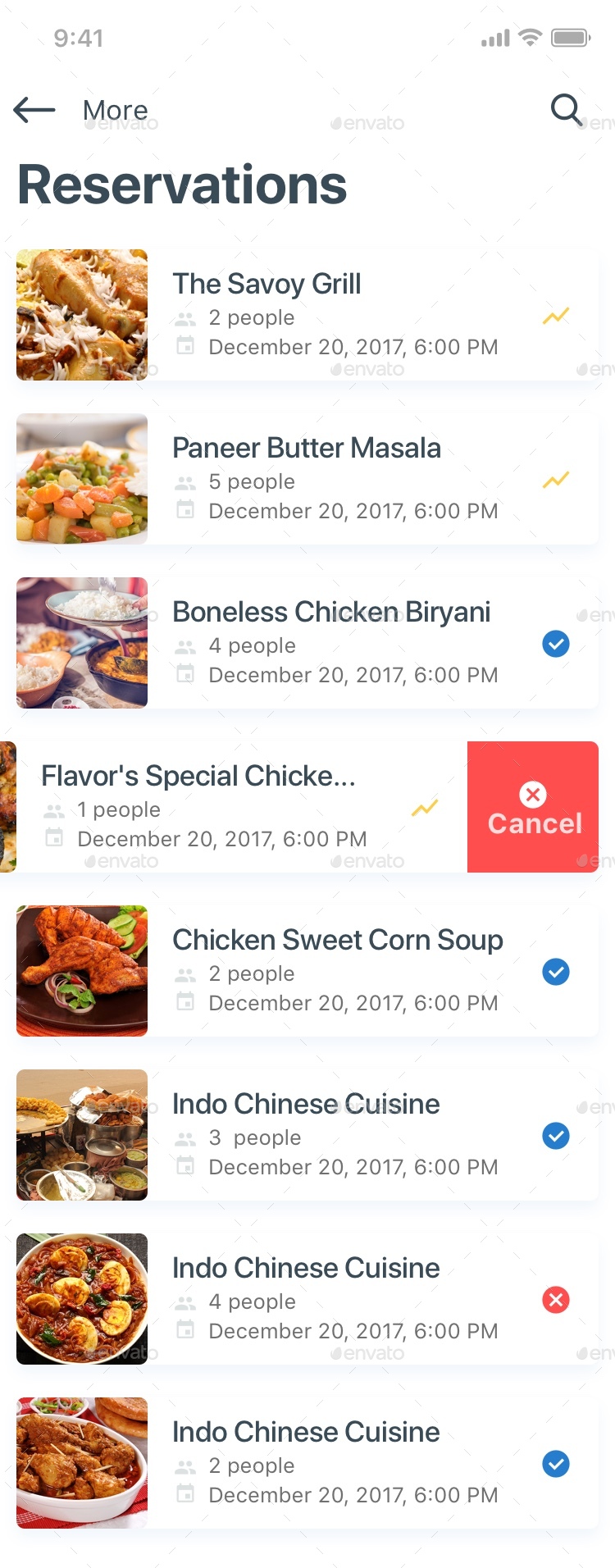Screenshot of a smartphone menu displaying reservations for various dishes. In the upper left corner, the time shows 9:41, and on the right side, icons indicate signal strength, Wi-Fi, and battery status. Below that, there is a search feature represented by a magnifying glass and an empty search bar. To the left, a button labeled "More" with an arrow pointing left is visible.

The main heading in large text reads "Reservations." Below this, a list of reservations is present:

1. **The Savoy Grill**
    - Reservation for two people on December 20, 2017, at 6:00 PM.
    - On the left, there is an image of a dish that appears to be chicken topped with shredded cheese.

2. **Paneer Butter Masala**
    - Reservation for five people on December 20, 2017, at 6:00 PM.
    - On the left, a dish featuring orange and green vegetables is visible.

3. **Boneless Chicken Biryani**
    - Reservation for four people on December 20, 2017, at 6:00 PM.
    - An image of the dish is shown on the left.

4. **Flavors Special Chicken** (partially cut off)
    - On the right, there is a red "Cancel" button.
    - A list of four additional food items follows:
        - The bottom item has a blue check mark next to it.
        - The item above it has a red dot.
        - The next two items above have blue check marks.
        - A "Cancel" button in red is noted just above these items.

This detailed menu provides a clear view of various dinner reservations with images and descriptions of each dish.